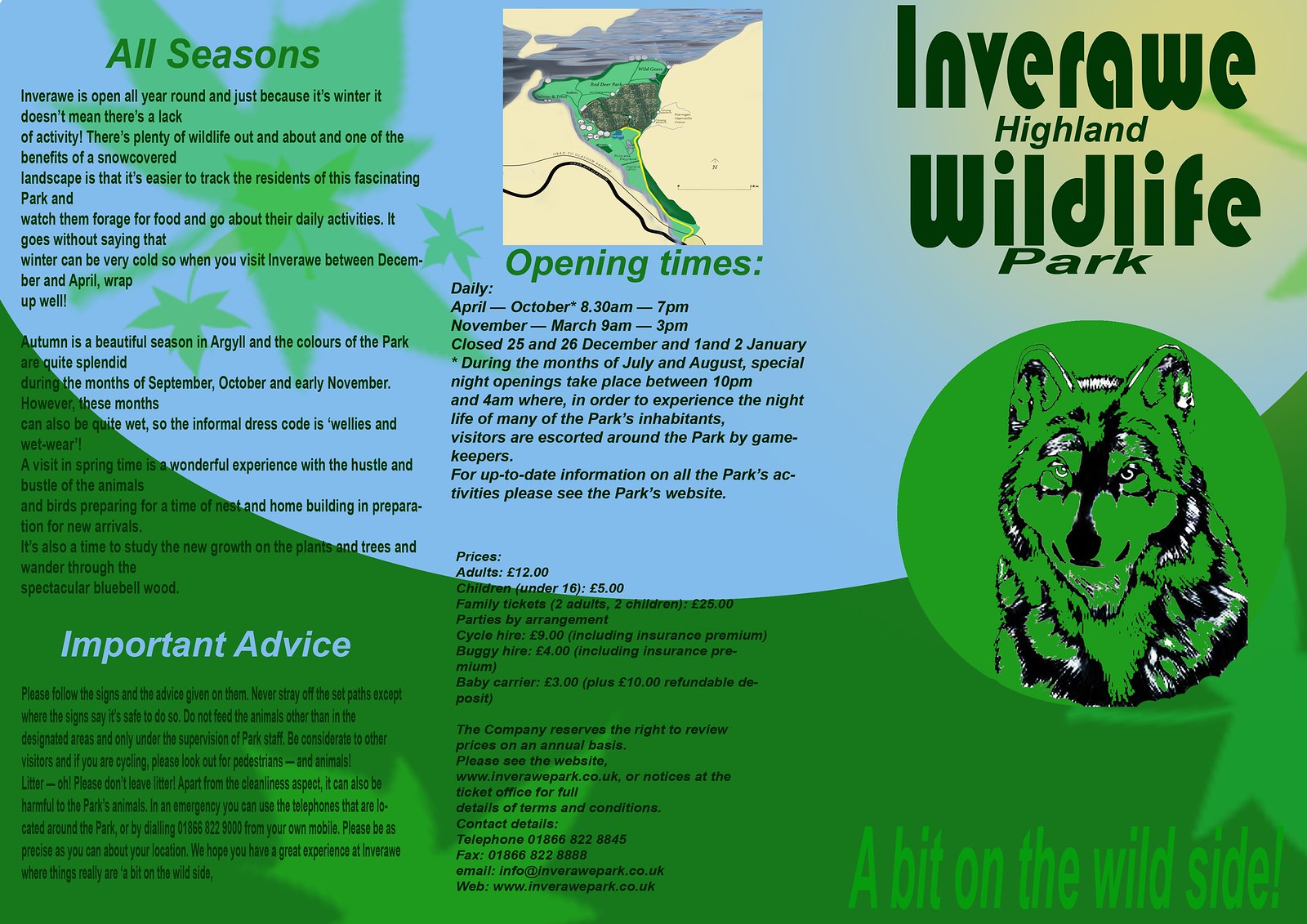This pamphlet for the Inverraw Highland Wildlife Park is divided into three sections, featuring a harmonious blend of natural hues, such as blue skies, green grass, and decorative leaves. The left section, titled "All Seasons" in bold green writing, emphasizes that the park is open year-round and highlights various seasonal activities. It provides detailed information on wildlife activities during winter and autumn, explaining how snow makes tracking the park's residents easier. Below this section, "Important Advice" is highlighted in large light blue letters, offering essential tips and guidelines for visitors.

The middle section features a map of the park at the top, showcasing various attractions and pathways within the wildlife sanctuary. Just below this, it mentions "Opening Times," listing the operational hours from April to October and noting the days the park is closed in November. Further down, it provides the admission prices: adults at 12 pounds, children under 16 at 5 pounds, and family tickets at 25 pounds.

The right section prominently displays the park's name, "Inverraw Highland Wildlife Park," with "Inverraw" and "Wildlife" in larger, dark green font, while "Highland" and "Park" are in smaller green text. Below the name, there is a circular logo featuring an illustration of a wolf in green and black. At the bottom, the phrase "A Bit on the Wild Side!" in lighter green is superimposed on the grassy background, drawing attention to the park's adventurous appeal.